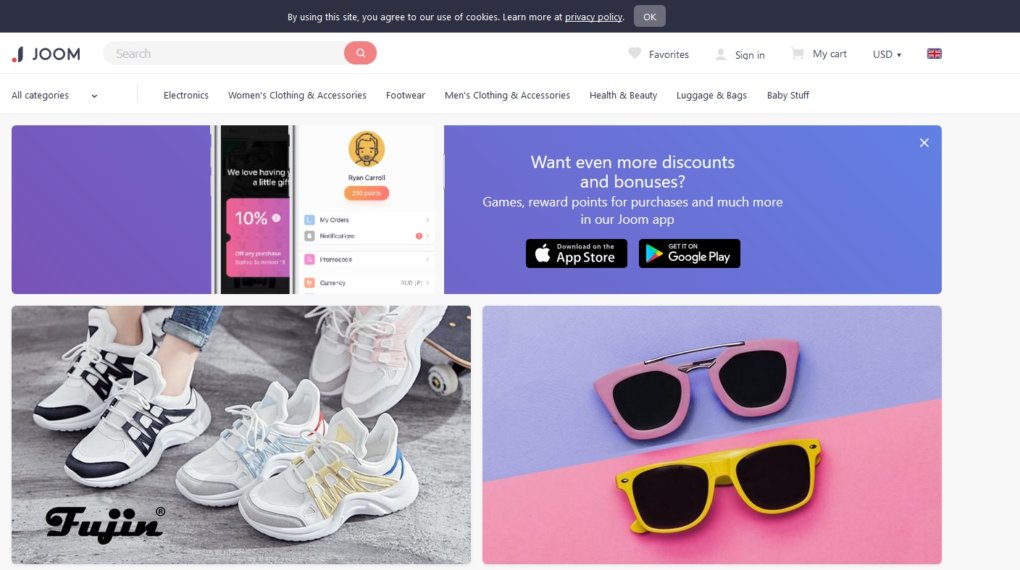The image showcases the homepage of the e-commerce website Joom. At the very top of the page, a black notification bar spans the width of the screen with the message: "By using this site, you agree to our use of cookies. Learn more at Privacy Policy" (underlined). To the right of this message is a gray button with the word "OK" in white text.

Below the notification bar, the website's header section features a white background. On the left side, the brand name "Joom" is prominently displayed in bold letters. To its right, a light gray search bar includes the placeholder text "Search" and is accompanied by a pink search button with a magnifying glass icon.

Further to the right of the search bar, a series of icons and text provide quick access to various site functions: "Favorites" with a heart icon, "Sign In" with a user silhouette, "Cart" with a shopping cart icon labeled "My Cart," and a currency selector denoted by "USD" with a dropdown menu and a Union Jack flag to indicate the current currency.

Immediately below the header is a navigation menu bar that includes dropdown options and links to different product categories: "All Categories," "Electronics," "Women's Clothing," "Accessories," "Footwear," "Men's Clothing and Accessories," "Health and Beauty," "Luggage and Bags," and "Baby Stuff."

Occupying the main content area below the navigation menu are four distinct sections. The first section on the left features user account and settings options, listing items such as "Ryan Carroll," "My Orders," "Notifications," "Preferences," and "Currency." Below these options is an offer or message that is partially visible, mentioning something about loving gifts and indicating a 10% discount.